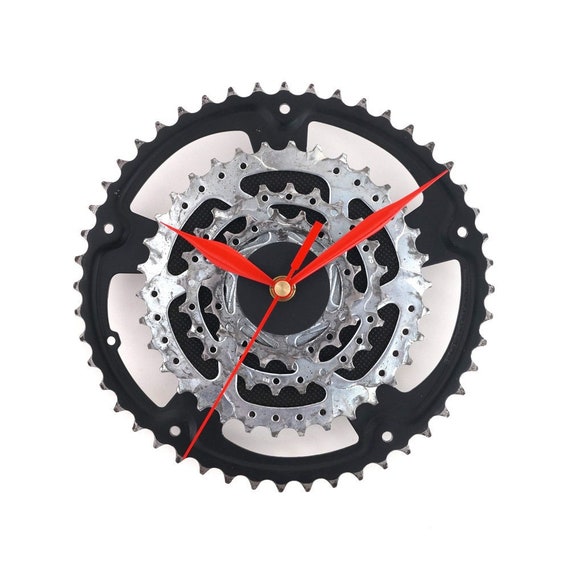This color photograph features a square-format depiction of a clock ingeniously crafted from bicycle gears. The outer gear ring, which is black and has five spokes extending to the center, encases a series of silver gears stacked in descending size. These gears serve as the backdrop for the clock hands, which are all red. The hour hand points to 10 o'clock, the minute hand is at 10 minutes past the hour, and the second hand is positioned around the 7 o'clock mark. Central to this composition is a gold stud securing the clock hands. The entire object appears to be floating against a stark white background, emphasizing the clock’s intricate design. The photographic style is representational, focused on realism and precise product photography.